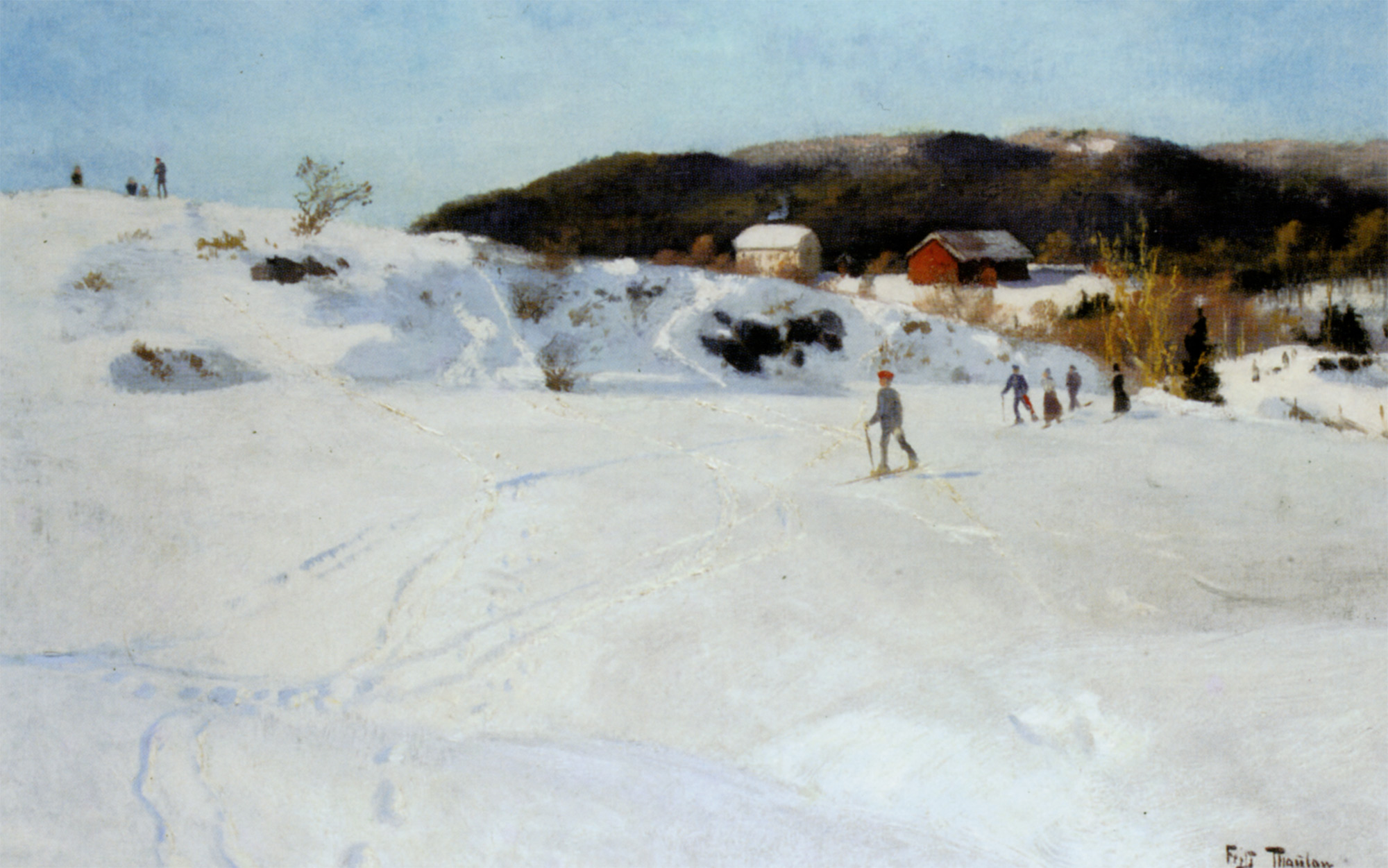The painting captures a serene winter scene set against a pale baby blue sky. A rolling snow-covered landscape dominates the foreground and mid-range, detailed with ski tracks. Among the hills, a family of cross-country skiers traverses the heavy snowpack, their figures faint and dressed in turn-of-the-century attire, identifiable by their poles but lacking intricate details. The background features a rural setting with a three-story house emitting chimney smoke, indicating a cozy fire within, accompanied by a large red barn. Trees and plants scatter around a lower valley, while dark, snow-touched mountains rise in the distance, partially covered in green foliage. Five indistinct figures are visible on a snow ridge to the left, appearing as small black dots, suggesting human activity. The artwork is signed with an illegible scrawl in the bottom right corner. The palette includes shades of white, green, brown, red, blue, gray, and yellow, emphasizing the wintry beauty and tranquility of the rural landscape.